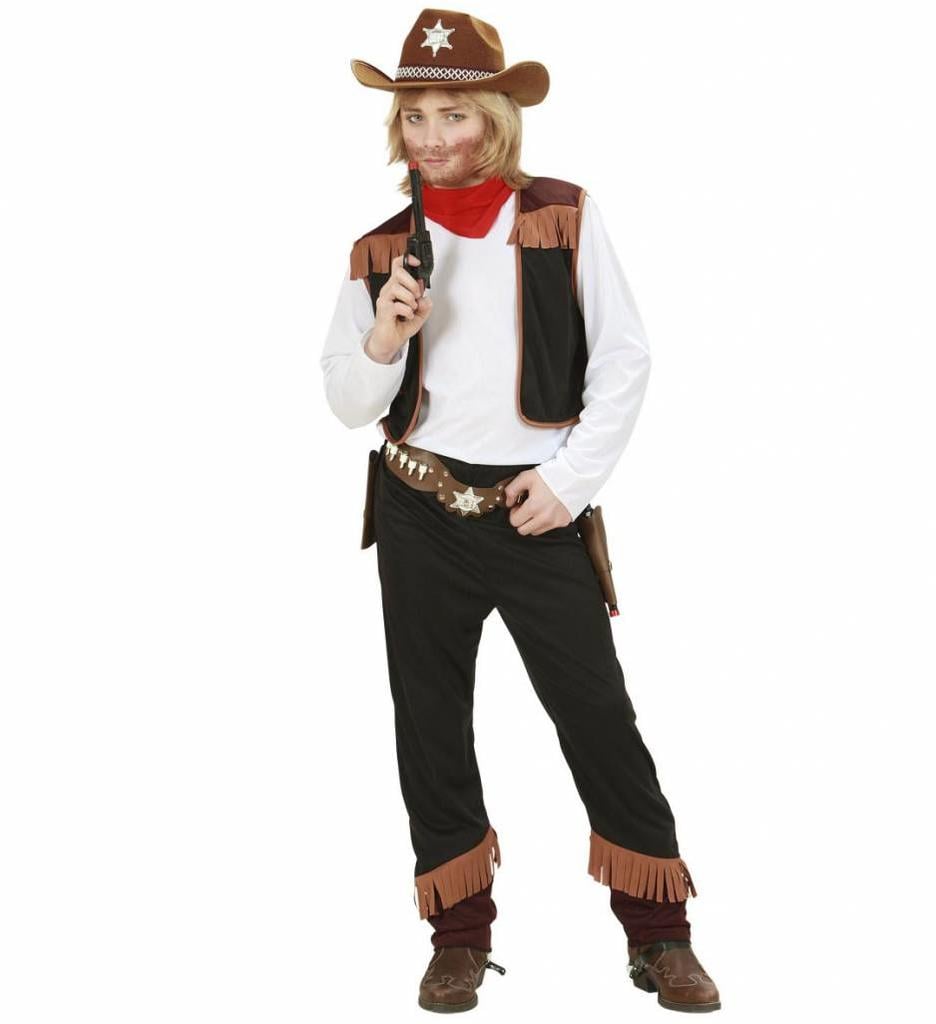This image captures a model dressed in a cheaply mass-produced cowboy Halloween costume. The model, possibly a young woman with a drawn-on beard and blonde hair, wears a brown cowboy hat adorned with a silver sheriff's star. She accessorizes with a small red bandana around her neck and a white silky shirt under a tight brown vest featuring tassels on the shoulders. Pointing a fake black gun with a red cap into the air with her right hand, she also has her left hand resting on a belt that sports another sheriff's star and a holster. Completing the outfit, she dons black pants with brown tassels at the bottoms and brown cowboy boots. The overall look is more theatrical and playful rather than practical or serious.